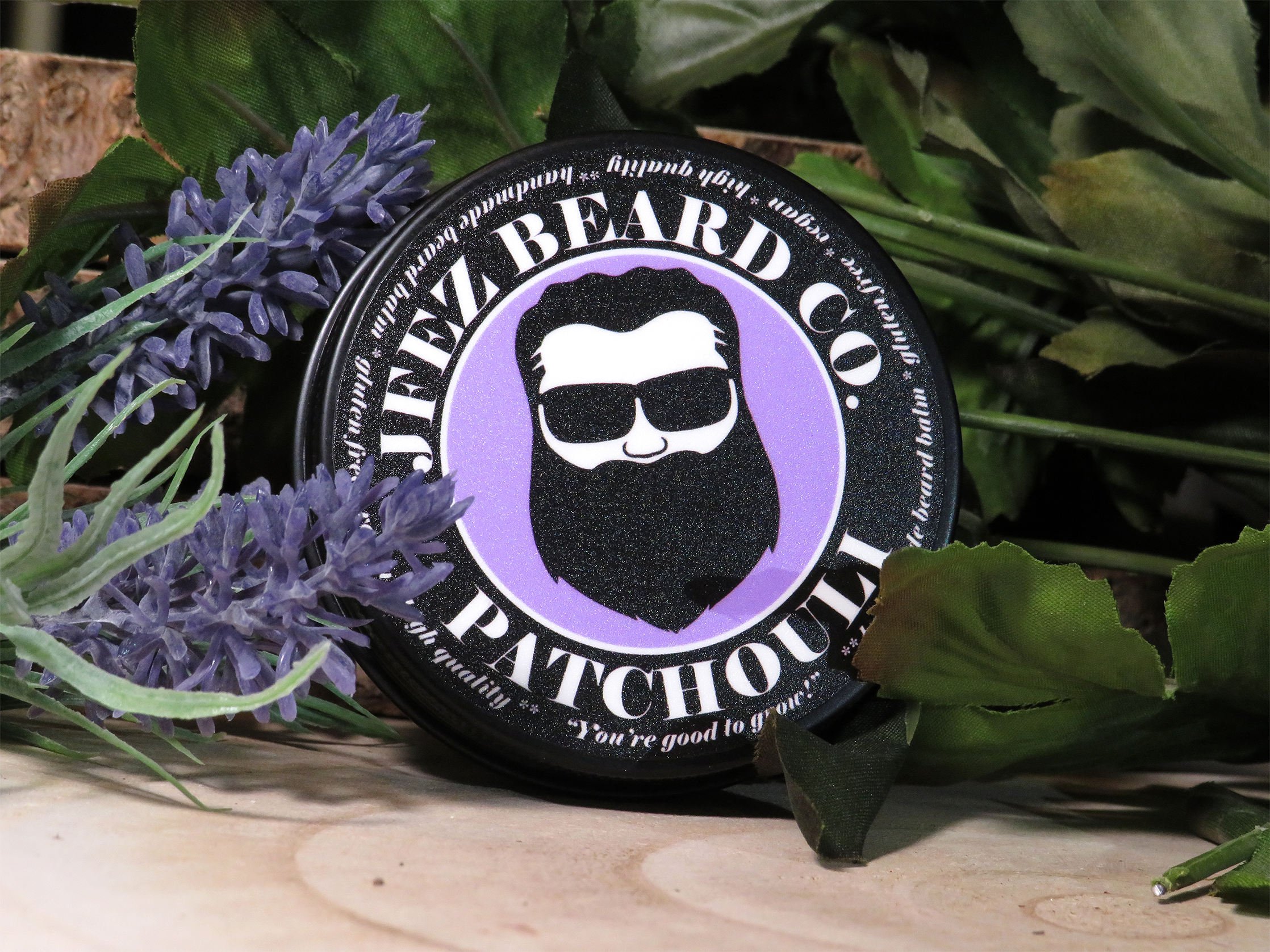In this photograph, a black, circular-shaped badge is prominently displayed on a light brown wooden plank surface. The center of the badge features a light purple circle containing a cartoonish silhouette of a man's face, adorned with a long beard and sunglasses. Surrounding this image, white text reads "G's Beard Co.," and below the central purple circle, it spells out "Patchouli" in capital letters. An additional quote in smaller text reads, "You're good to grow." To the left of the badge are two sprigs of lavender with purple flowers, while on the right side, there are dark green leaves. The scene captures an intriguing combination of natural elements, suggesting an outdoor setting, although the artificial appearance of the foliage hints it might have been taken indoors.